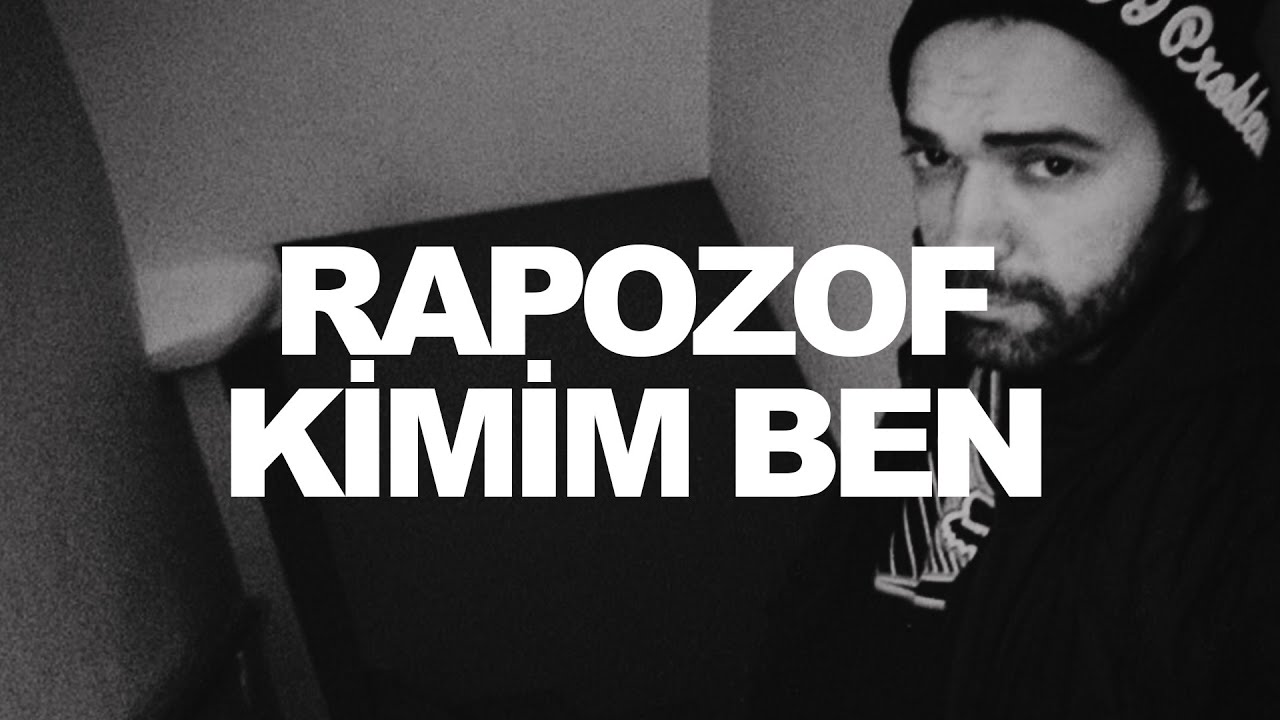In this black and white photograph, a young man with a thick beard and a neutral expression takes a selfie, standing on the right side of the image. He wears a dark beanie with partially legible white lettering that seems to spell out "problem." The man is dressed in dark clothing, including a black sweater and a t-shirt with a white graphic that is difficult to decipher due to the folds in the fabric. The background features a stark contrast with two walls converging and a very dark floor, possibly indicating he's in a stairwell or near a corner. Prominently displayed in the center of the image are large white block letters that read "RAPOSOV," followed by "KIMIM" and "BEN," with the I's in "KIMIM" appearing in a distinct lowercase style.